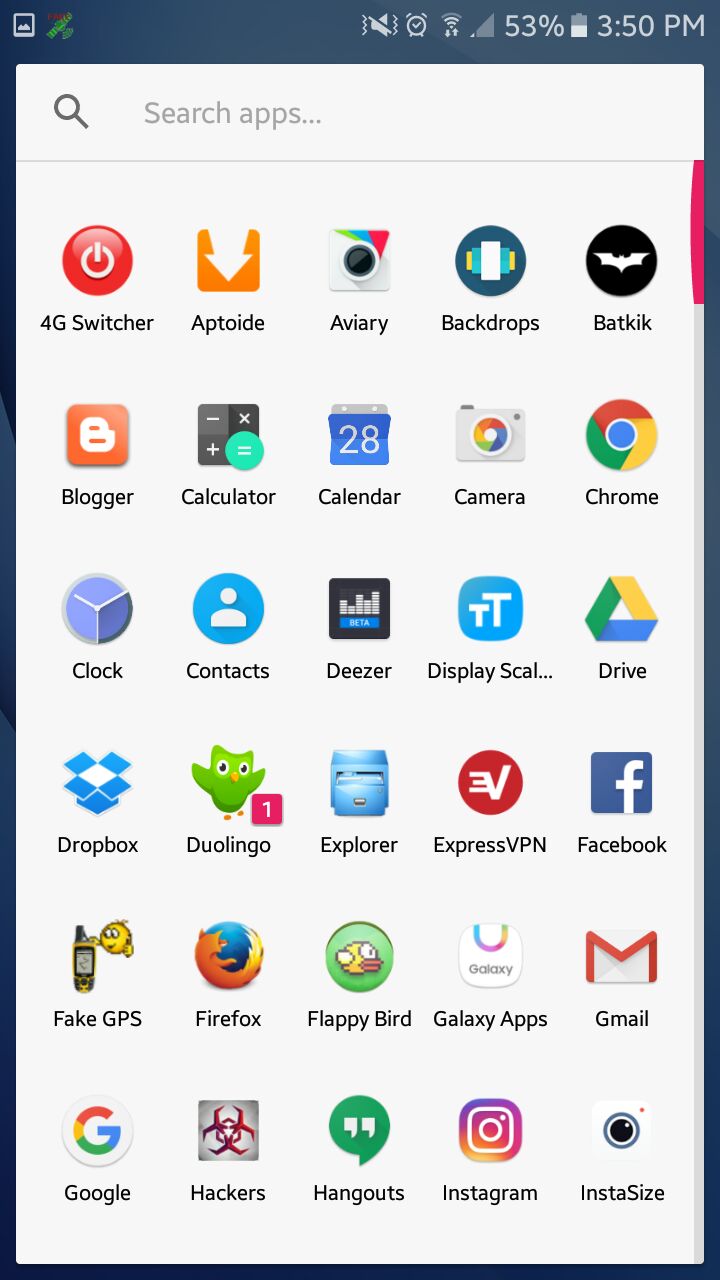The image appears to be a screenshot of a pop-up on a mobile device. The background is a navy blue color. On the left side, there is a gray square with a zigzag line, likely indicating an absent image or a recently taken photo. Adjacent to this, there's a green icon that resembles a satellite.

On the right side of the image, there's an icon of a crossed-out horn, flanked by two zigzag lines, that represents the vibrate mode. Next to it, there's an alarm clock icon, followed by a Wi-Fi signal icon showing poor reception. The battery icon is white and slightly more than halfway full, showing 53% charge. The time displayed is 3:50 PM.

Dominating the top part of the image is a gray pop-up rectangle. The upper section of this pop-up, in a darker gray, features a magnifying glass icon. This is followed by the lighter gray text: "Search apps...". Below this is a thin gray line delineating a section where various app icons are displayed in a grid format, with five apps per row and six rows in total.

The apps are listed as follows:

First row:
1. 4G Switching
2. Apple Toy
3. Aviary
4. Backdrop
5. Bat Cake

Second row:
1. Blogger
2. Calculator
3. Calendar
4. Camera
5. Chrome

Third row:
1. Clock
2. Contacts
3. Display Scal...
4. Drive

Fourth row:
1. Dropbox
2. Duolingo
3. Explorer
4. Express VPN
5. Facebook

Fifth row:
1. Fake GPS
2. Firefox
3. Flappy Bird
4. Glassy Apps
5. Gmail

Sixth row:
1. Google
2. Hackers
3. Hangouts
4. Instagram